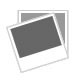In this horizontal rectangular image, a person's left hand is prominently displayed, holding a large, jagged piece of white crystalline rock. The rock, possibly quartz, glistens in the sunlight, highlighting its shiny, almost transparent quality. It is mostly white, but features streaks of gray and black near its base. The background is blurred, showcasing lush greenery, which seems to be a pine tree with visible pine needles. In the upper left corner of the image, yellow text indicates "14," followed by dimensions of "5 by 4 by 2.5 inches," and a weight of "1.1 pounds," likely describing the size and weight of the rock.